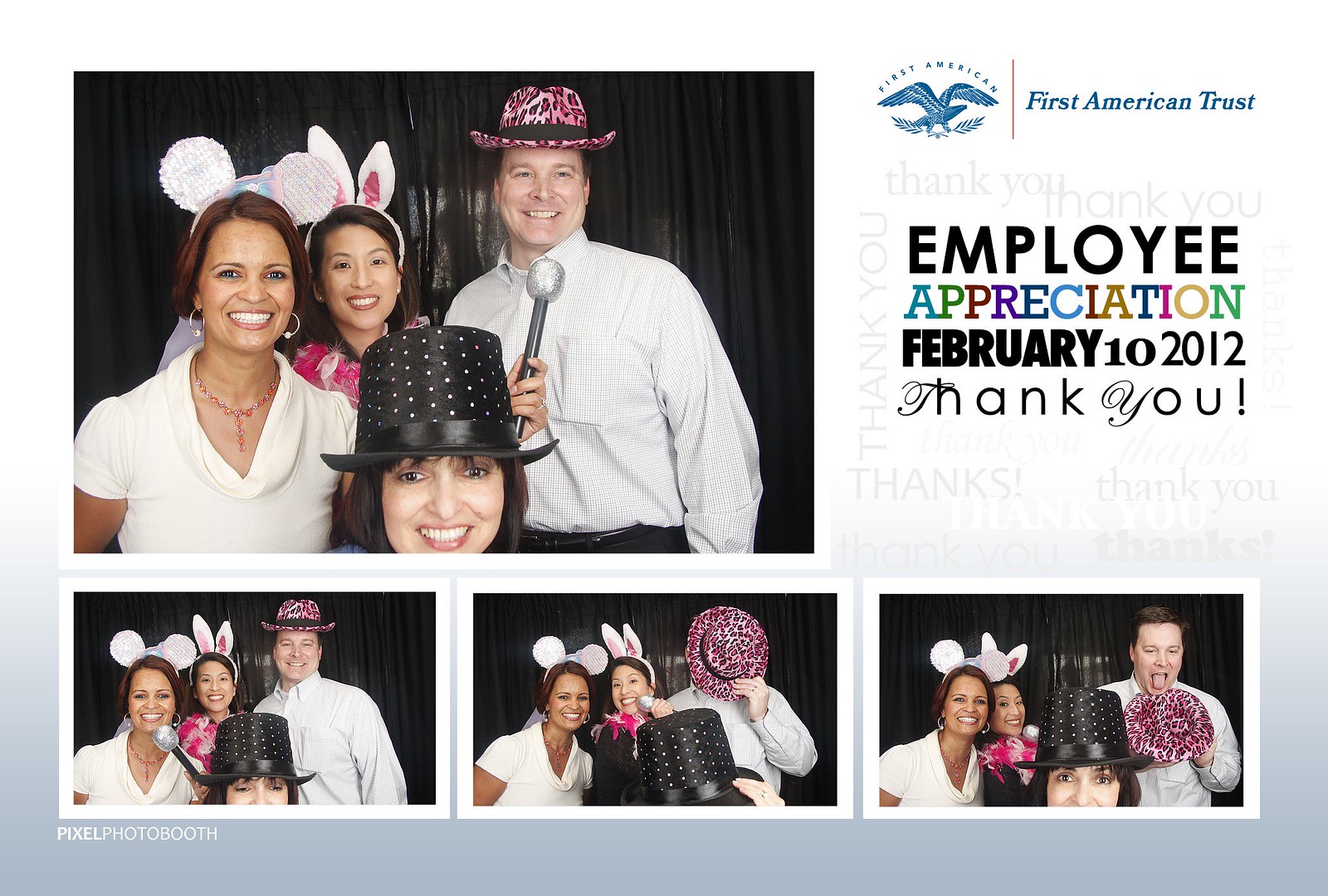The image is a photo booth collage from the First American Trust Employee Appreciation event on February 10, 2012. The background transitions from white to light gray. The central, largest photograph, located at the upper left, features four people standing against a black backdrop. Dominating the foreground is a close-up of a woman wearing a black top hat adorned with white polka dots. Behind her, on the left, is a woman in a white shirt with sequin Mickey Mouse-style ears and another woman with white rabbit ears. To the right stands a man wearing a pink and black leopard print cowboy hat. The upper right corner of the image showcases the First American Trust logo, featuring an eagle carrying olive branches, alongside text that reads, "First American Trust Employee Appreciation February 10, 2012." Below the central photograph are three smaller pictures, each displaying the same four individuals in various poses, continuing to wear their distinctive hats and headbands. The overall design is complemented by a repeated background of "thank you" in gray.